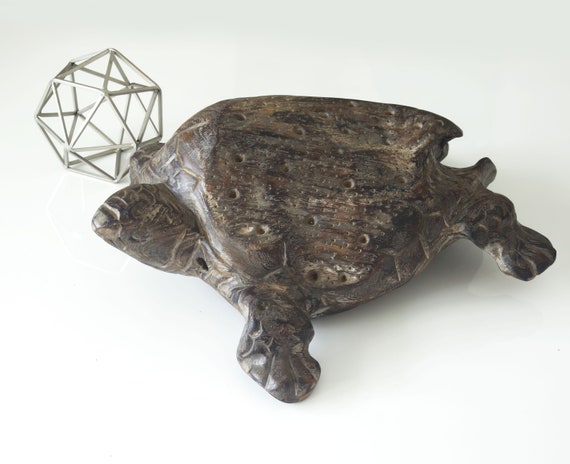The photograph features a rough wooden sculpture of a sea turtle set against a solid white background. The sculpture, which has a weather-worn appearance, is carved to resemble a turtle facing to the left of the image. Its shell showcases natural flaws and imperfections in the wood, including a notable missing chunk at the back where the turtle's tail might be. The turtle's feet are represented by notches, and its shell is marked by several small, partial drill holes. Adjacent to the turtle, positioned towards the upper left of the image, is a 20-sided, hollow metal sculpture. This geometric piece is composed of triangular facets, bearing a resemblance to a skeletonized decahedron, and adds a contrasting metallic element to the overall composition.